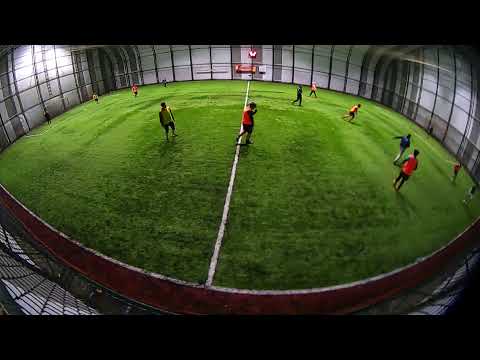The image captures an indoor soccer practice session at a smaller training facility with no spectators, featuring approximately a dozen players. The field appears worn and is likely covered with green astroturf bordered by white lines, including a dividing stripe down the middle. The facility has arching walls that extend upwards, partially visible with white and gray hues. A brown perimeter surrounds the field. Key figures include a person in a red shirt and black shorts near the central dividing line, another in a green shirt and black shorts to the left, and someone in a red outfit, with red and black pants, while another individual wears blue and white pants on the right. Shadows suggest overhead lighting. The image is bordered by thick black lines at the top and bottom, framing the panoramic scene.